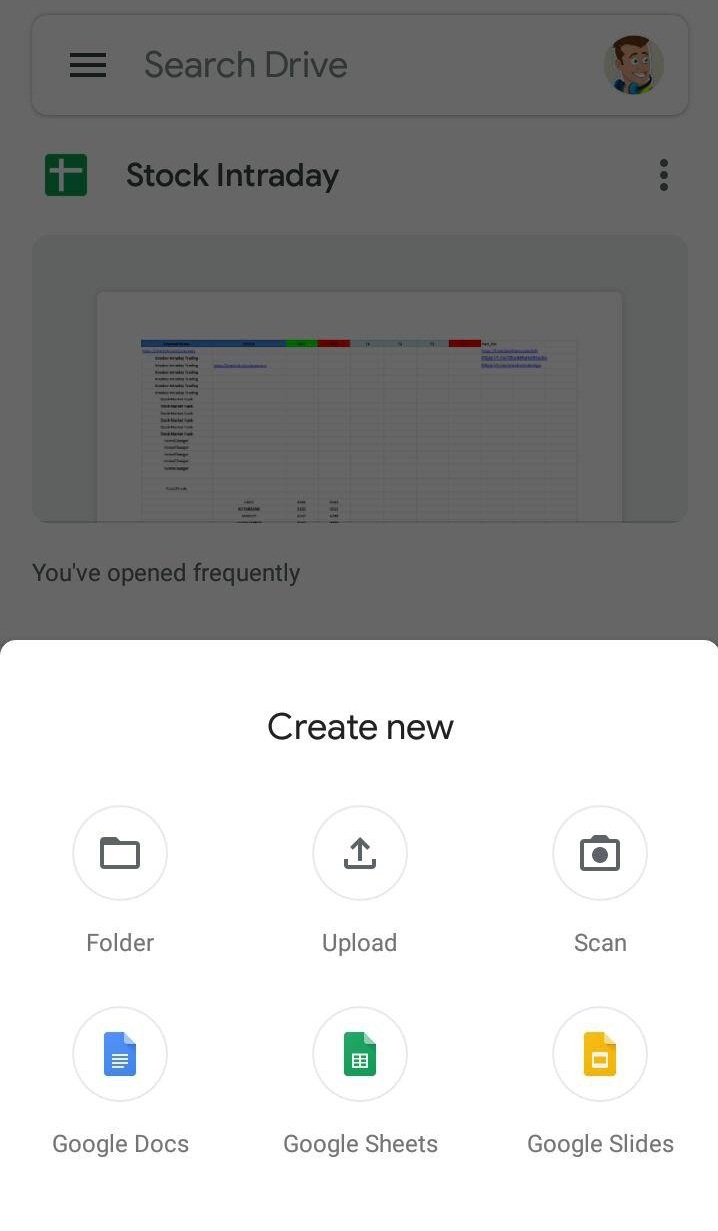At the top of the image, there is a grayed-out white bar containing a search feature. On the left side of this bar, there are black lines, indicating the search icon. Inside the search bar, it reads "search drive" in gray text. To the right side, there is a picture of a cartoon character representing the user's profile image. The character appears to be a white person looking to the right.

Beneath this top bar, on a white background, there is a gray and green square featuring a white cross in its center. Next to this square, the text "stock intraday" is written. On the right-hand side of this section, there are three vertical dots, indicating additional options or a menu.

Below this section, there is what appears to be an Excel spreadsheet, filled with various cells containing different colors. Underneath this, the text "you frequently opened" is displayed.

Centrally located towards the bottom of the image, on a white background, the phrase "create new" is presented in black text. Beneath this phrase, there are three buttons arranged horizontally. The first button has an icon of a folder with the label "folder" below it. The second button features an upvote icon with the label "upvote". The third button bears a camera icon labeled "scan".

Additionally, there are icons of a blue paper, a green paper, and a yellow paper. These represent "Google Docs," "Google Sheets," and "Google Slides," respectively, with each icon labeled accordingly below it.

The remainder of the image does not contain any additional information pertinent to the description.